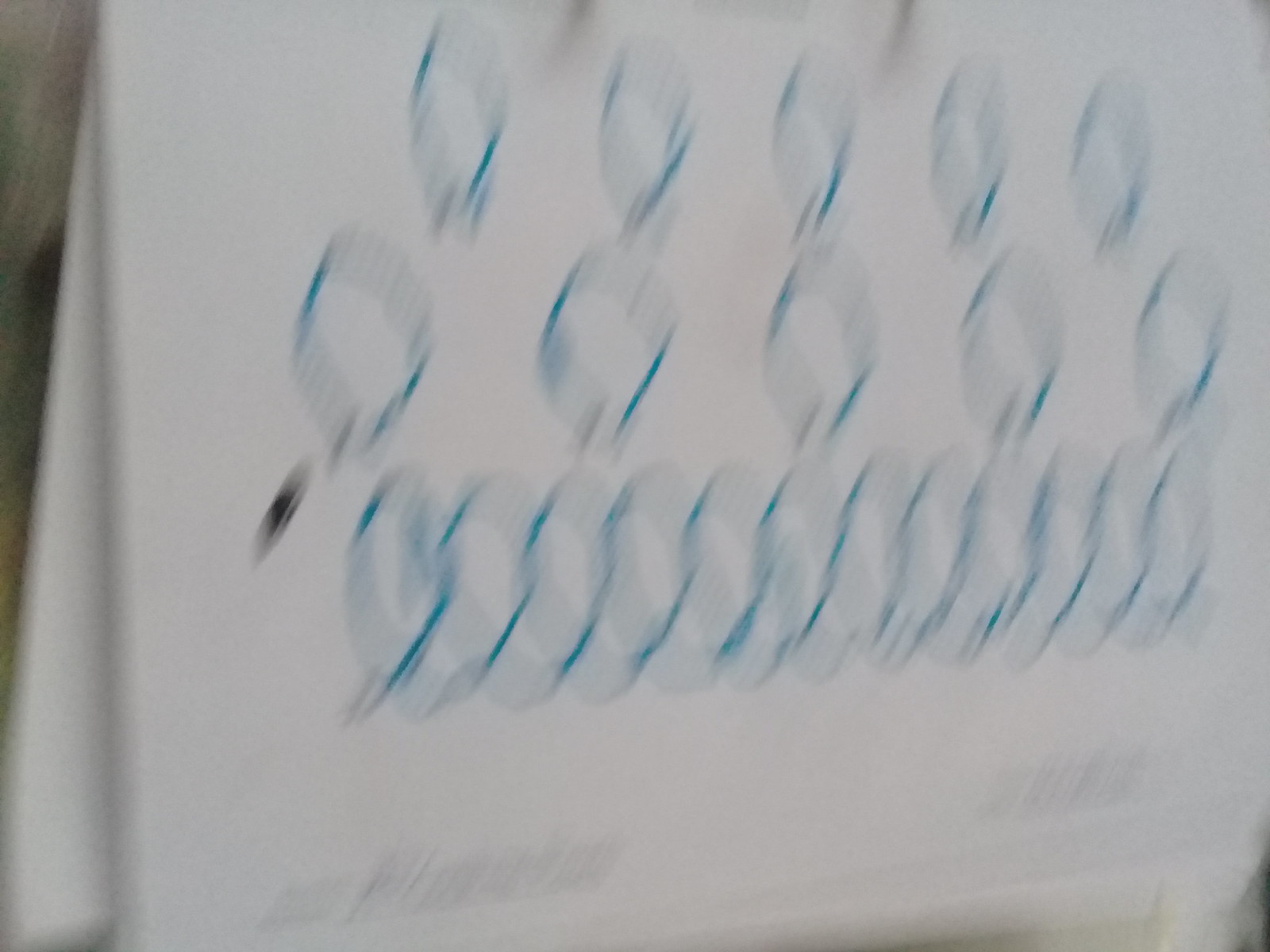The image depicts a very blurry, white poster board or similar large sheet, with a folded section partially visible behind it. Covering the white surface are several blue shapes resembling narrow, upside-down horseshoes or circles with two solid vertical lines followed by wavy lines. The top row features five distinct blue shapes, followed by another row of five equally spaced shapes beneath them. Below these rows, a horizontal line of approximately thirteen connected blue shapes can be seen, though they're overlapping and the image lacks clarity. There's also a noticeable black fuzzy mark near the upper left region of the third row. The entire composition is difficult to discern due to the image's blurry quality and zoomed-in perspective.